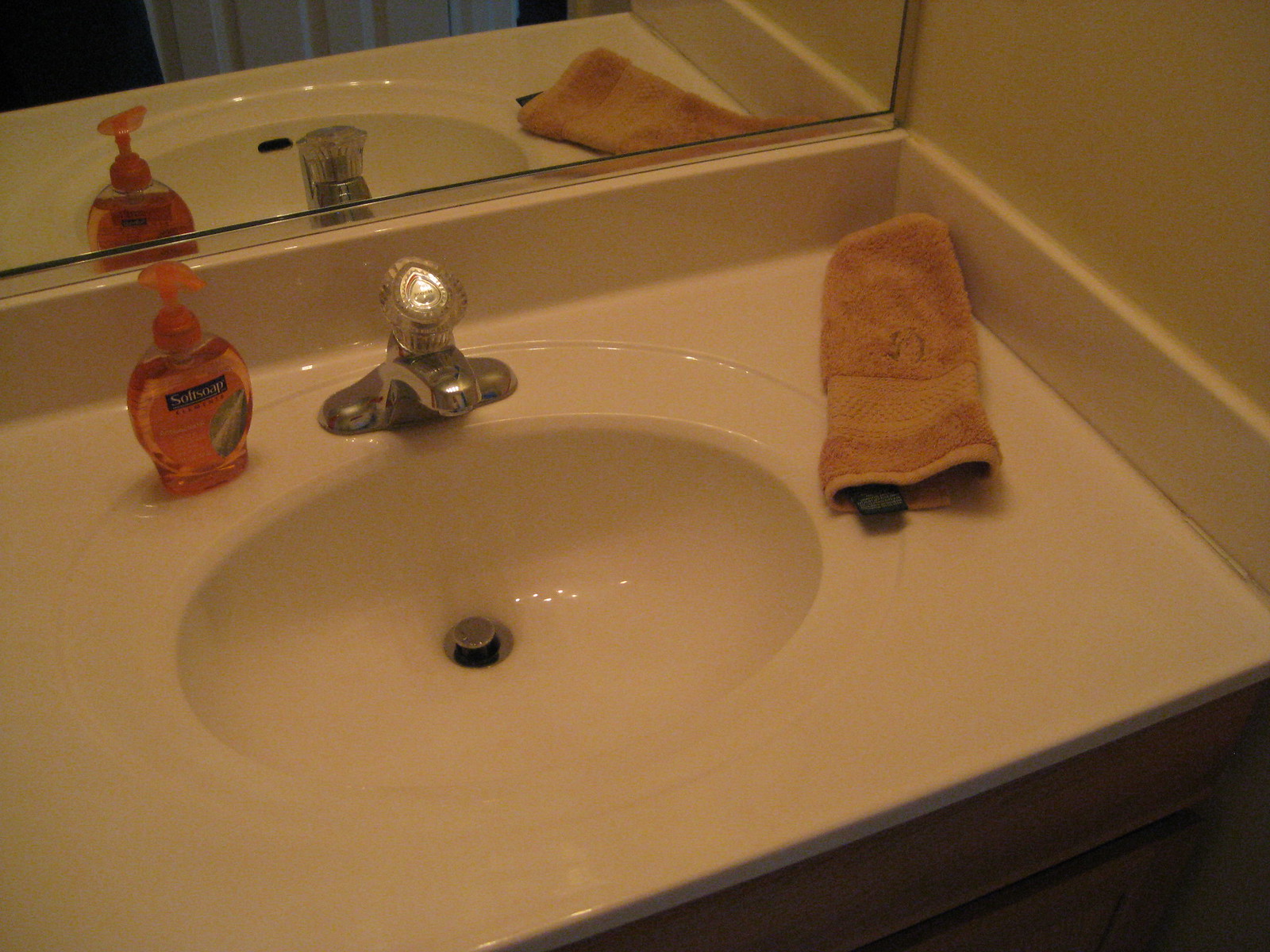A dimly lit bathroom corner is captured in this simple yet detailed photograph. At the center is an off-white or white sink with a single faucet fixture featuring a clear plastic dial controlling hot and cold water. The faucet is positioned towards the upper left corner of the image. To the left of the faucet is an orange bottle of soft soap. A peach-colored hand towel is neatly folded and placed at a diagonal into the corner of the sink unit. The sink is perfectly nestled into a nook in the wall, creating a cozy and functional space. Above the sink, a mirror is partially visible, adding depth to the scene. The sink unit itself appears to be made of brown wood, with parts of it visible in the lower right corner of the photo.